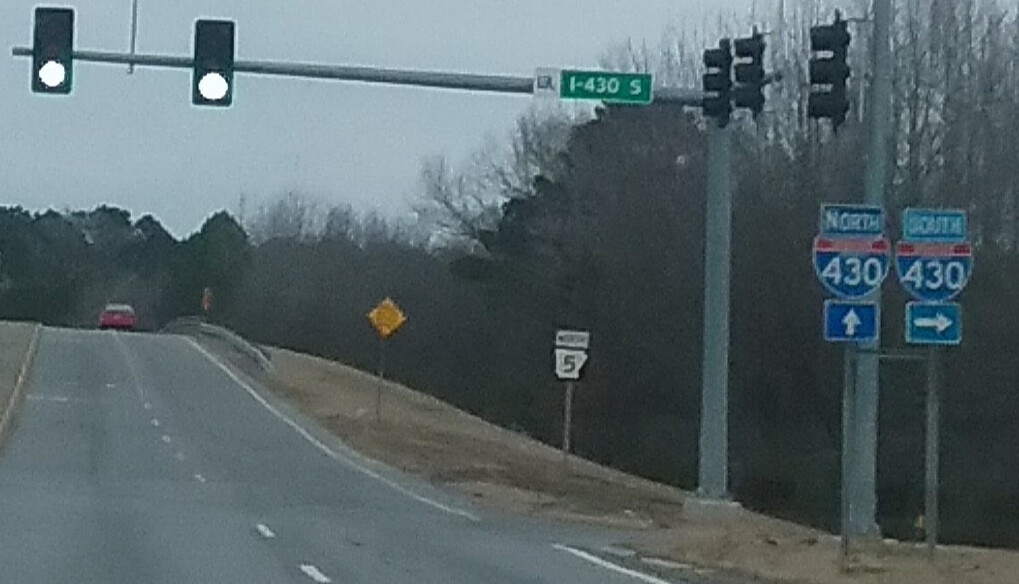An outdoor color photograph captured during dusk or on a heavily overcast day depicts a scene of a two-lane highway extending northward. Overhead, two streetlights illuminate the road, casting a faint glow in the dim light. Attached to a sign on the right side of the road, a green traffic light signals go, hanging over the roadway. The sign itself displays "I-430S", directing drivers, with three other streetlights oriented in the opposite direction.

On the roadside to the right, two interstate signs guide travelers: one indicates "North 430" with an arrow pointing straight ahead, and the other displays "South 430" with an arrow directing to the right. These signs are prominently colored in blue, red, and white lettering, characteristic of interstate markers. 

Additionally, a road sign stands by the lane marked "North 5". In the distance, slightly out of focus, the rear of a small red car can be seen traveling northward along the highway, contributing a sense of motion and direction to the tranquil scene.